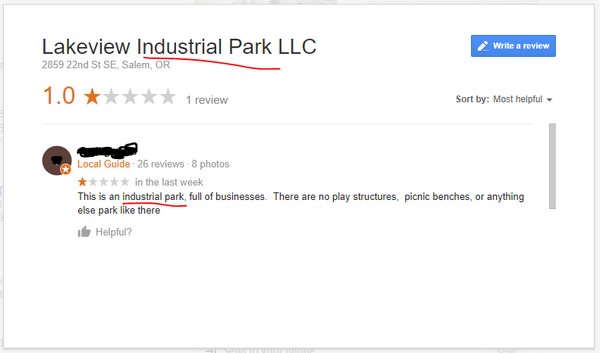The image depicts an online review site for businesses. The background is predominantly white. On the top left corner, the business name "Lakeview Industrial Park LLC" is displayed along with its address, "2859 22nd Street Southeast, Salem, Oregon," all in gray text. Below the address, the business has a rating of 1.0 displayed in orange, accompanied by one orange star and four gray stars, and the text "one review" next to it in gray.

In the upper right corner of the image, there is a small blue rectangle featuring a pencil icon and the text "Write Review" in white. Below this section, there is a sorting option indicated by the phrase "Sort by: Most Helpful" with an accompanying small upside-down triangle.

The main review area features a user thumbnail that is partially obscured, showing only brown and black colors. Next to it, a name is scribbled out and labeled as "Local Guide" in orange. The user has "26 reviews, 8 photos" written in gray text below their title. The user's review is marked with one orange star and four gray stars, indicating the user's rating given in the last week.

The content of the review reads: "This is an industrial park full of businesses. There are no play structures, picnic benches, or anything else park-like here."

At the bottom of the review, there is a thumbs-up icon with the word "Helpful" in gray followed by a question mark.